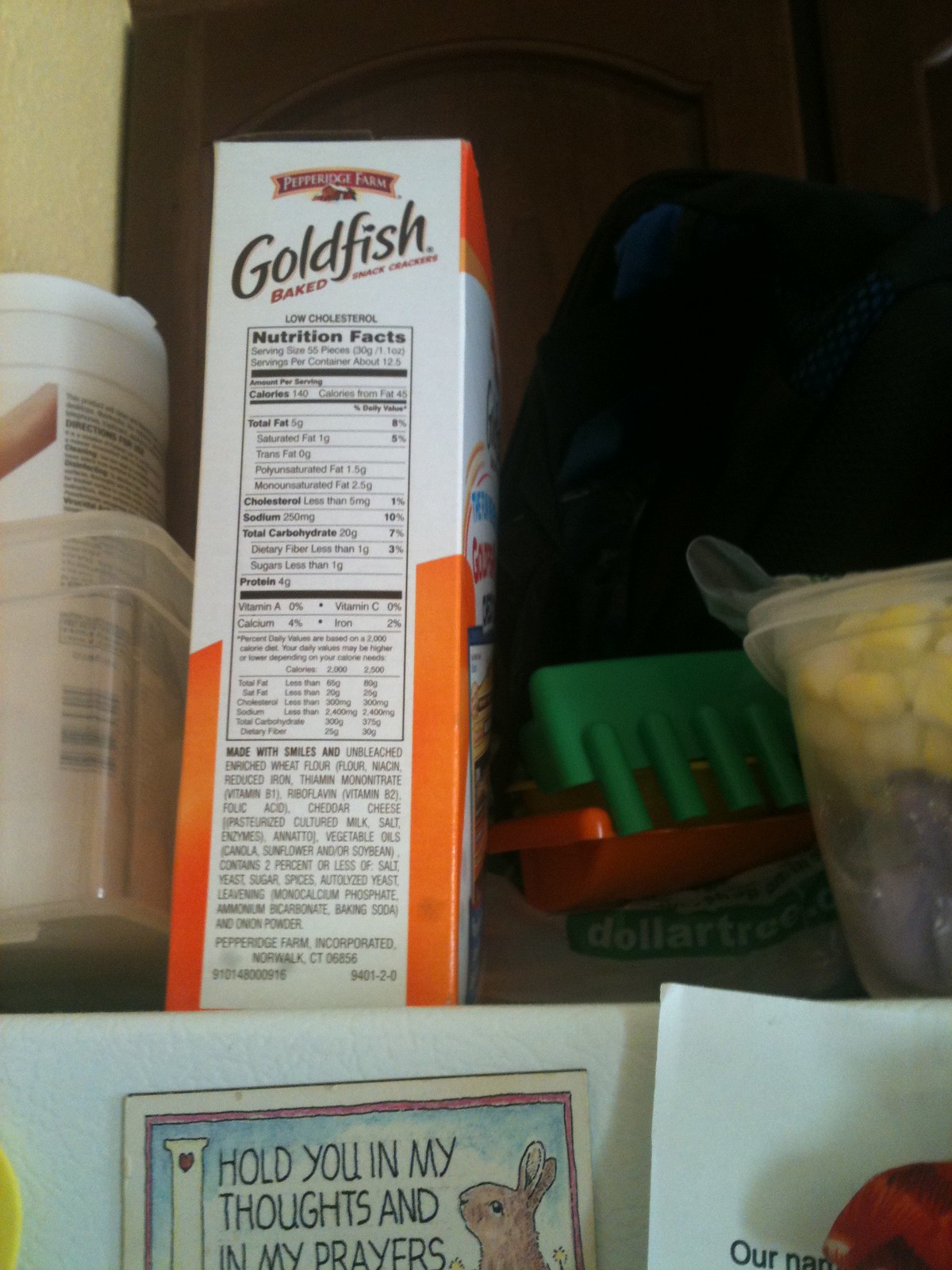This photograph captures a cluttered space in a kitchen, focusing on various items on a shelf located on top of a refrigerator. The central element in the image is the side of a box of Pepperidge Farm Goldfish baked snack crackers, prominently displaying its nutrition facts and details about low cholesterol and ingredients. Flanking the box is a transparent plastic container housing other white and brown containers, hinting at additional stored items, possibly snacks. Among the clutter, there are more stacked plastic containers and a plastic box. Attached to the shelf is a heartfelt card that reads, "I hold you in my thoughts and in my prayers," adorned with a small bunny rabbit illustration framed in pink over a blue background. In the backdrop, dark brown cabinets are faintly visible, contributing to the kitchen setting. Adjacent to the refrigerator is a Dollar Tree bag containing beach toys. A paper and a magnet, which features the same heartfelt message and bunny image, are affixed to the refrigerator door, drawing the eye to the personal touches in this domestic space.